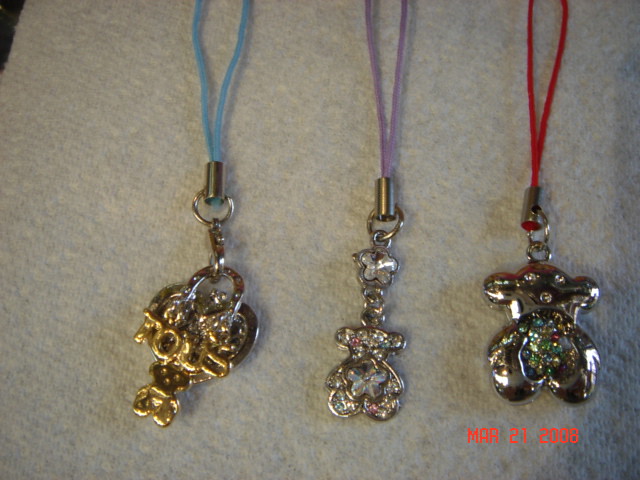This image captures three distinctive pendants, each adorned with unique features and colored strings, set against a gray fabric background. The pendant on the left features the letters "T.O.U.S." and is accented with gold plating. It hangs from a bright blue string. The middle pendant, shaped like a teddy bear, is the smallest and richly decorated with pink, blue, and green gems. It includes a tiny flower and is suspended from a vivid purple string. The pendant on the right, also a teddy bear, is primarily silver with gems embellishing its eye, nose, and stomach areas. It is attached to a vibrant red string. The timestamp "March 21st, 2008" is visible in the bottom right corner of the image.